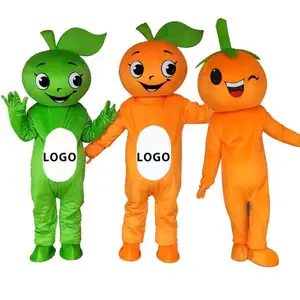This is a detailed product image of three mascot costumes designed to resemble fruit characters, set against a transparent background. From left to right: The first costume is a vibrant green, depicting a lime with a fruit-shaped head crowned by a leaf and stem, and a full body covered in green fur. The second costume in the center represents an orange fruit, featuring a round head with a similar leaf and stem, an entirely orange body, and an elliptical white patch on its belly that says "LOGO" in black letters, indicating customization options. The third costume on the right is also orange, sporting a tall stem on top of its head, a cheerful smile with a playful wink, and a full orange fur body. Notably, this costume does not have a "LOGO" patch on its front. The three figures appear friendly and inviting, perfect for mascot purposes.